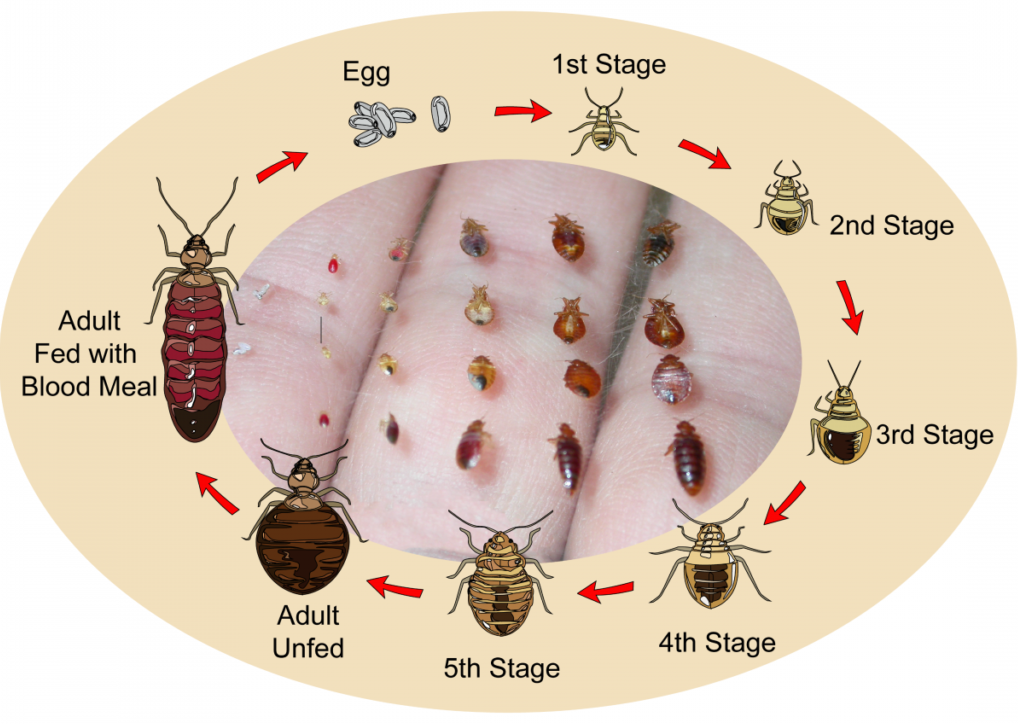This image showcases a detailed illustration and photograph of an insect's life cycle, likely depicting either ticks or bed bugs. The composition is oval-shaped, wider than it is tall, and features a prominent light brown or tan circle around the central photograph. The photograph in the center shows a close-up of someone's three fingers, each covered with numerous tiny bugs neatly arranged.

Around the perimeter of the circle, starting from the top left and moving clockwise, are labeled illustrations depicting the various life stages of the insect. It begins with an "egg" stage, followed by successive stages labeled as first, second, third, fourth, and fifth stages. The depiction continues with the "adult unfed" stage, where the insect's body is wider than long, culminating at the "adult fed with blood meal" stage, where the insect's body appears elongated and reddish, signifying that it has consumed a blood meal.

Each stage is interconnected by arrows, detailing the insect's transformation from one stage to the next, eventually completing its life cycle.